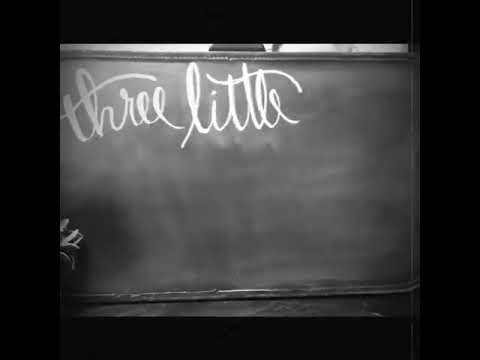The black and white image prominently features a chalkboard that fills almost the entire frame. The chalkboard has a wooden border, though its exact color is indeterminate due to the monochromatic nature of the photo. Written in a detailed, flourished cursive script at the top left corner of the chalkboard are the words "Three Little." These words are composed with notable embellishments, especially the T's which have elaborate crossbars. The chalkboard itself appears clean aside from this text. In the lower left corner, there is a faint, ambiguous shape that resembles a hand but is difficult to identify clearly. The photo also suggests that the chalkboard might be placed on an easel, with the stand faintly visible at the top of the image. The left side of the frame hints at the presence of a partially visible plant in a vase, adding a subtle, additional element to the scene.